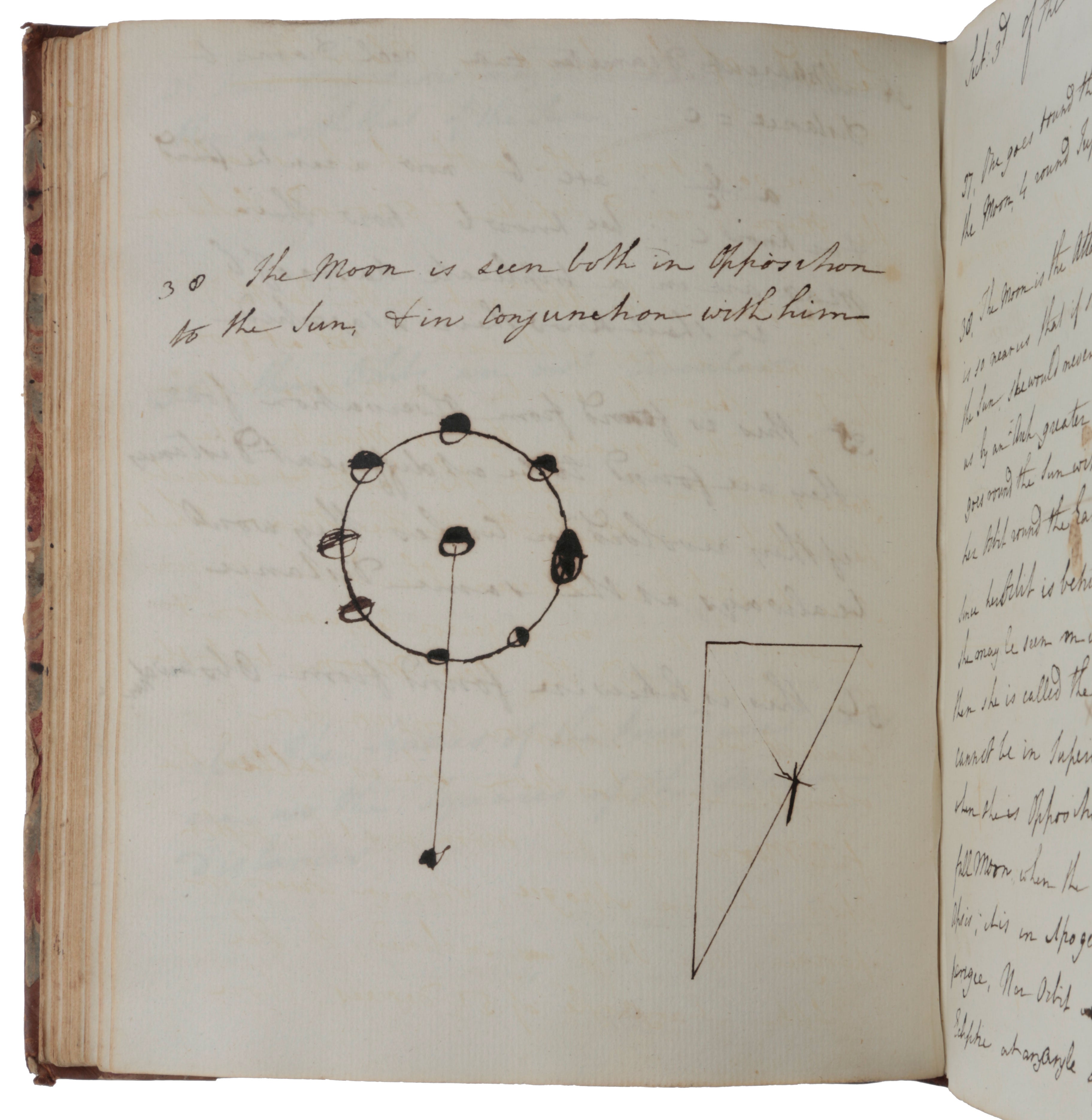This photograph depicts an open journal with a white background, showing predominantly the left-hand page while the right-hand page is turned upwards and mostly out of frame, making its content hard to discern. The left page, which appears to be somewhere in the middle of the book, is covered in neat handwriting. The most legible text reads, "The moon is seen both in opposition to the sun and in conjunction with him." Nearby, the text "3-0" is visible. The page also features a detailed diagram with a circle at the center, possibly illustrating the moon phases, showing a blackened area representing the dark side of the moon and a white area indicating the illuminated part. Radiating from the center is a line intersecting the larger circle, suggesting some celestial calculations or representation. To the right of this diagram is a triangle, which has been noted to include a right angle and possibly depicts angles of 60 degrees and 30 degrees, suggesting some geometric or astronomical context. Some areas of the page show signs of bleed-through or overlapping ink from adjacent pages.